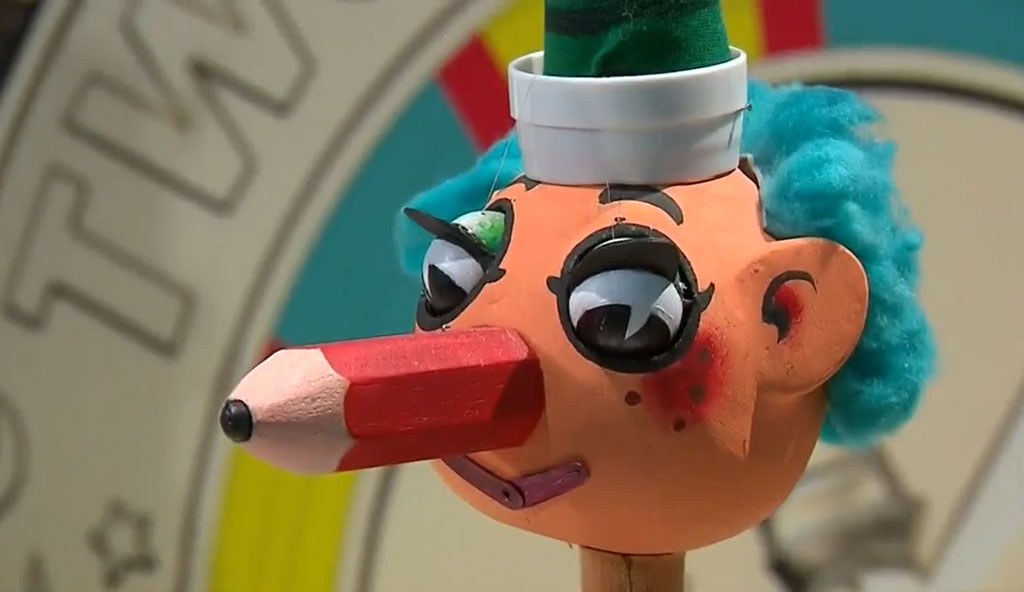The image depicts a whimsical, clay-like doll's face set against a colorful, blurred background. The doll has a peach-colored complexion and large eyes with black pupils and green eyelids, accented by black eyelashes and brown freckles below them. The mouth resembles two dark red, popsicle-stick-like strips. Its nose is a red wooden pencil with a tan sharpened tip and a black lead point. The doll sports fuzzy, teal cotton-like hair and wears a hat that appears as a white base with a green cone extending from the top, resembling a flower pot. The background features a blend of yellow, blue, red, white, and black colors, adding a vibrant contrast to the artwork. The image is horizontally oriented, capturing the doll from the neck up and revealing a partially obscured circular object with some writing, displaying visible letters "T" and "W" amidst colors of yellow, teal, and red.